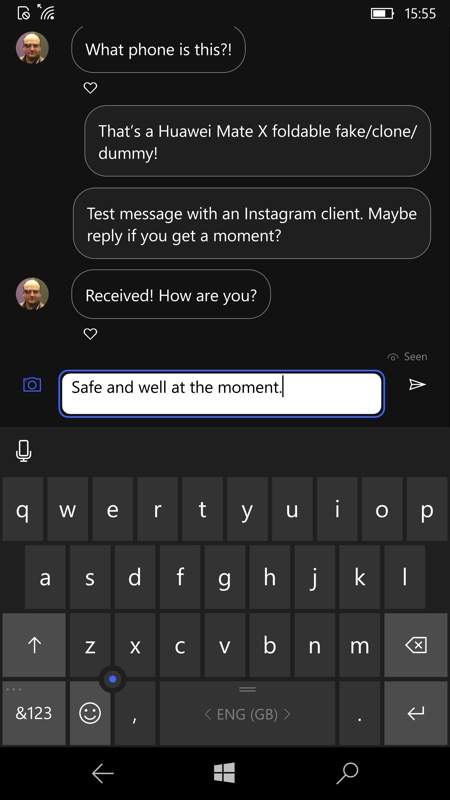In the image, a conversation between two users is depicted with the first user's messages on the left side and the main user's on the right. The background of the conversation is black, and the profile picture of the first user on the left is a photo of a man. The conversation starts with the first user asking, "What phone is this?" in white text. Below this, there is a heart reaction indicating their engagement with the message. 

The main user responds with, "That's a Huawei Mate X, foldable, fake or clone or dummy. Text messages, text message with an Instagram client, maybe reply if you get a moment." Following this, the first user acknowledges with "Received, how are you?" Notably, the text indicates that it has been seen, as stated at the bottom right side with "seen."

In the middle of the phone screen, there's a conversation box with a white background, black text, and a blue outline. This box also includes a blue camera icon on the left and a white send icon on the right. The text in the conversation box reads, "Safe and well at the moment," and shows an active cursor. Below, there is a keyboard featuring a white microphone icon on the top left for recording, along with a black background and black keycaps with white characters.